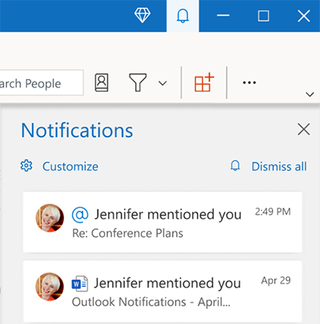Here's a detailed and cleaned-up caption for the described image:

---

The image is a screenshot from a smartphone displaying a user interface. At the very top, the screen has a blue border. In the upper-right corner, there are several white icons arranged in a row: a white 'X', the outline of a square, a white minus sign, a filled square, and a blue notification bell icon. To the left of the notification bell, there's a white diamond shape set against the blue background.

Below this header, a very light (almost white) section contains a partially visible search bar where only the letters "A-R-C-H" of the word "search" are readable, written in gray. To the right of the search bar is a small icon representing people.

Further down, the background shifts to light gray. On the left side of this section, "Notifications" is written in blue, followed by "Customize" directly beneath it. On the right side, the blue notification bell icon appears again, accompanied by the text "Dismiss all."

Below this header are two notification rectangles. Both notifications feature the same profile image—a round photo of a white woman with short blonde hair styled in a pixie cut. Each notification includes an '@' symbol, suggesting a mention on a social media platform, likely Twitter (or X). The text reads "Jennifer mentioned you," followed by the time and the subject of the mention. The second notification bears a 'W' icon but contains the same message and format as the first one.